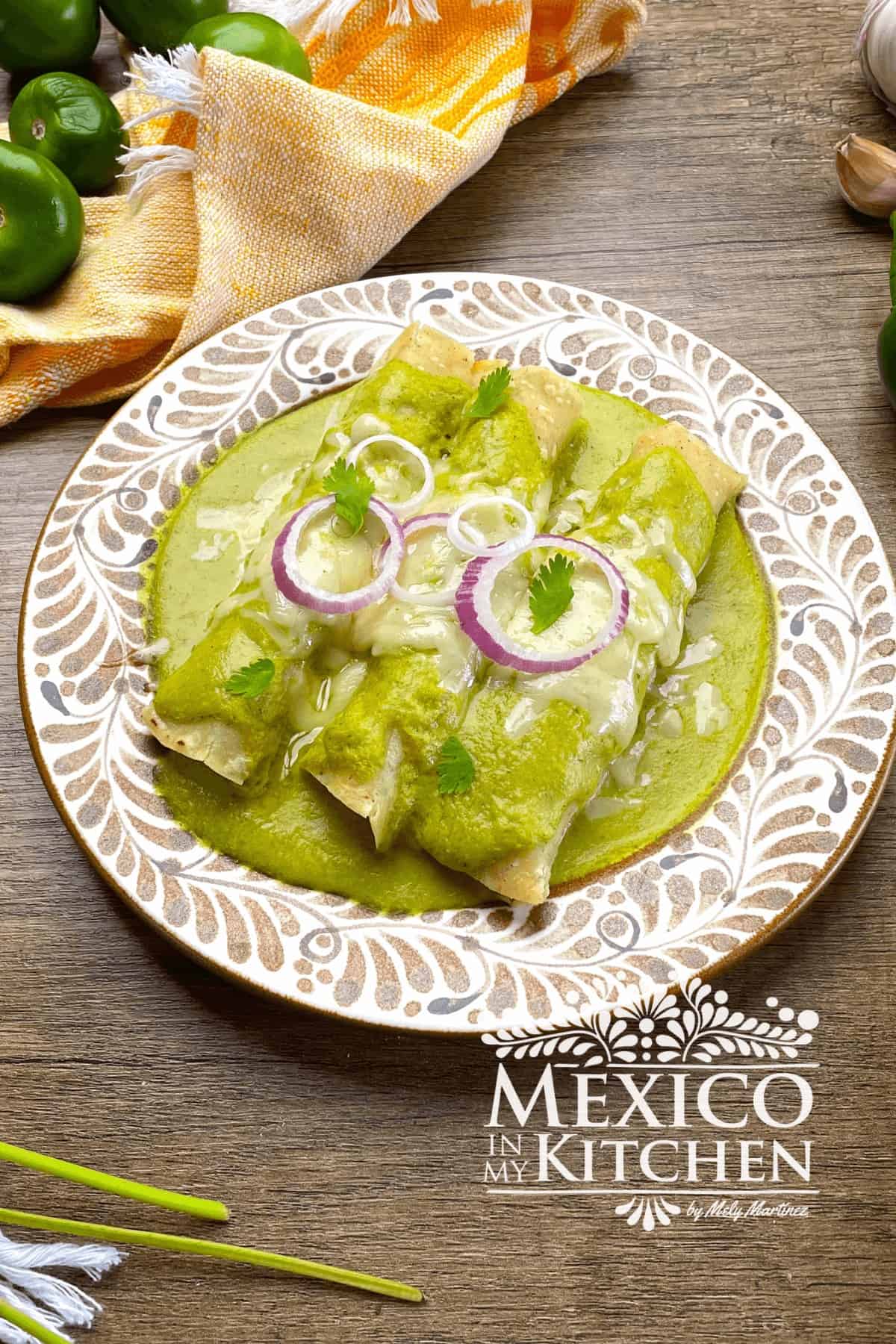This image is a detailed photographic illustration designed for "Mexico in My Kitchen" by Molly Martinez. It depicts a rustic scene on a dark-stained wooden table. At the top of the image, a richly colored orange dish towel is laid out with a few limes resting on it. The centerpiece is a white pottery plate accented with tan and gray designs, which holds three enchiladas generously covered in a vibrant green sauce, possibly avocado or a type of green salsa. The enchiladas are garnished with thinly sliced red onions and fresh cilantro leaves. Surrounding the plate are additional elements that enhance the authenticity of the scene: green peppers and cloves of garlic. The bottom right corner showcases the text "Mexico in My Kitchen" in elegant white font, accompanied by an ornate floral design with pre-Columbian influences, bringing a touch of cultural depth to the overall visual.